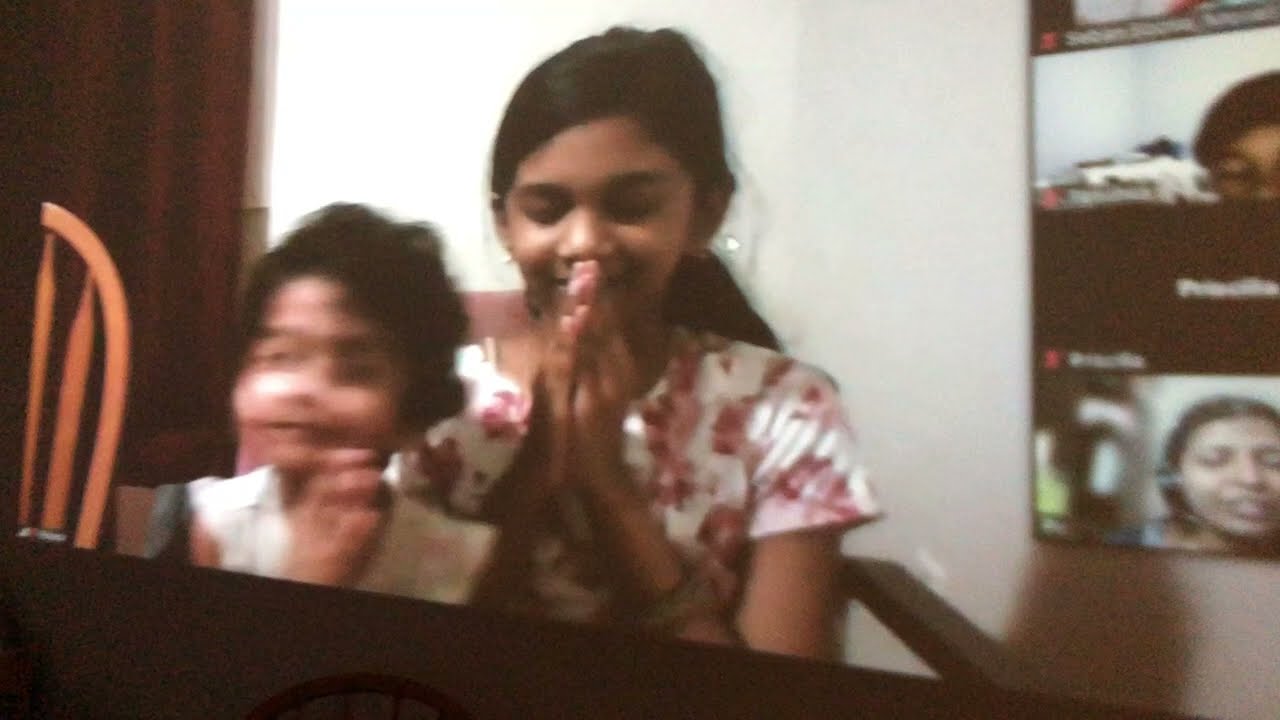The image depicts two children, one older girl and one younger boy, sitting at a black table in a room that appears to be either a kitchen or a living room. The older girl, slightly to the left of the image's center, has long black hair and wears a pink and white short-sleeved blouse with a red flower pattern. She sits with her hands in a prayer-like position just beneath her nose. Just below her right shoulder sits the younger boy, who has short dark hair and is wearing a white top. Both children are facing the camera. To the left, a brown rail-backed chair is partially visible. Behind the children, a white wall can be seen, and over the girl's left shoulder, a screen displays various faces from a Zoom call, highlighted with colors such as black from hair and red from the mute button. The overall focus of the image is somewhat blurry, particularly around the smaller child, causing their features to appear slightly misshapen.